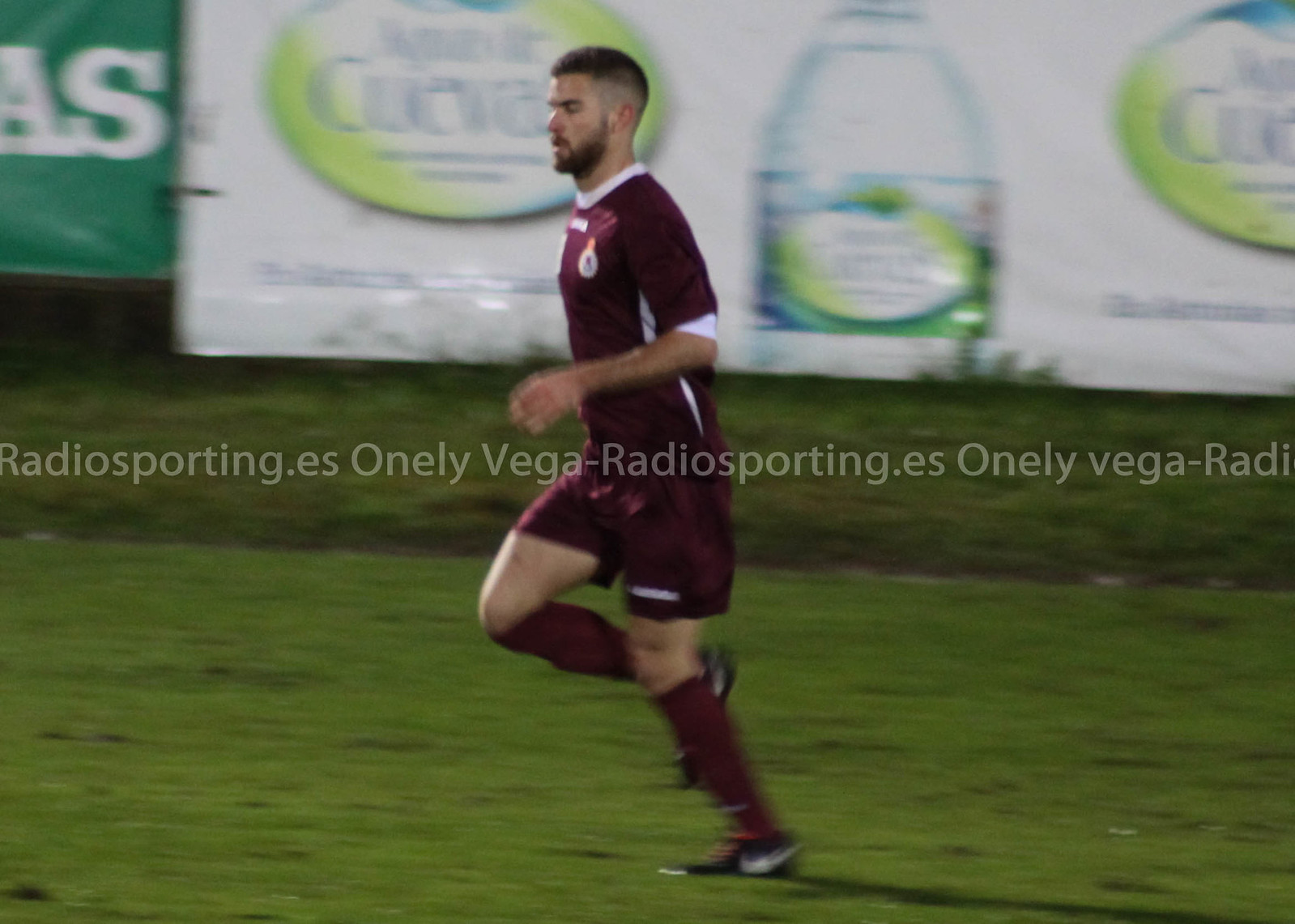The image captures a dynamic moment of a soccer player in action on a green field. The player, a gentleman with dark brown hair and a beard integrated with a mustache, is captured mid-run, with his right leg bent and lifted. He is attired in a maroon and white uniform: a maroon short-sleeved shirt with white accents on the collar, sides, and sleeves, paired with maroon shorts and socks. His feet are clad in black and white Nike sports shoes. Behind him, the scene is set against a backdrop of advertising banners. One banner prominently features a water bottle, while a green one displays partial text reading "AS." Another blurred banner stretches horizontally across the center, emblazoned with "radiosporting.es, Only Vega." The action and the vivid advertising elements hint at a lively outdoor match atmosphere.